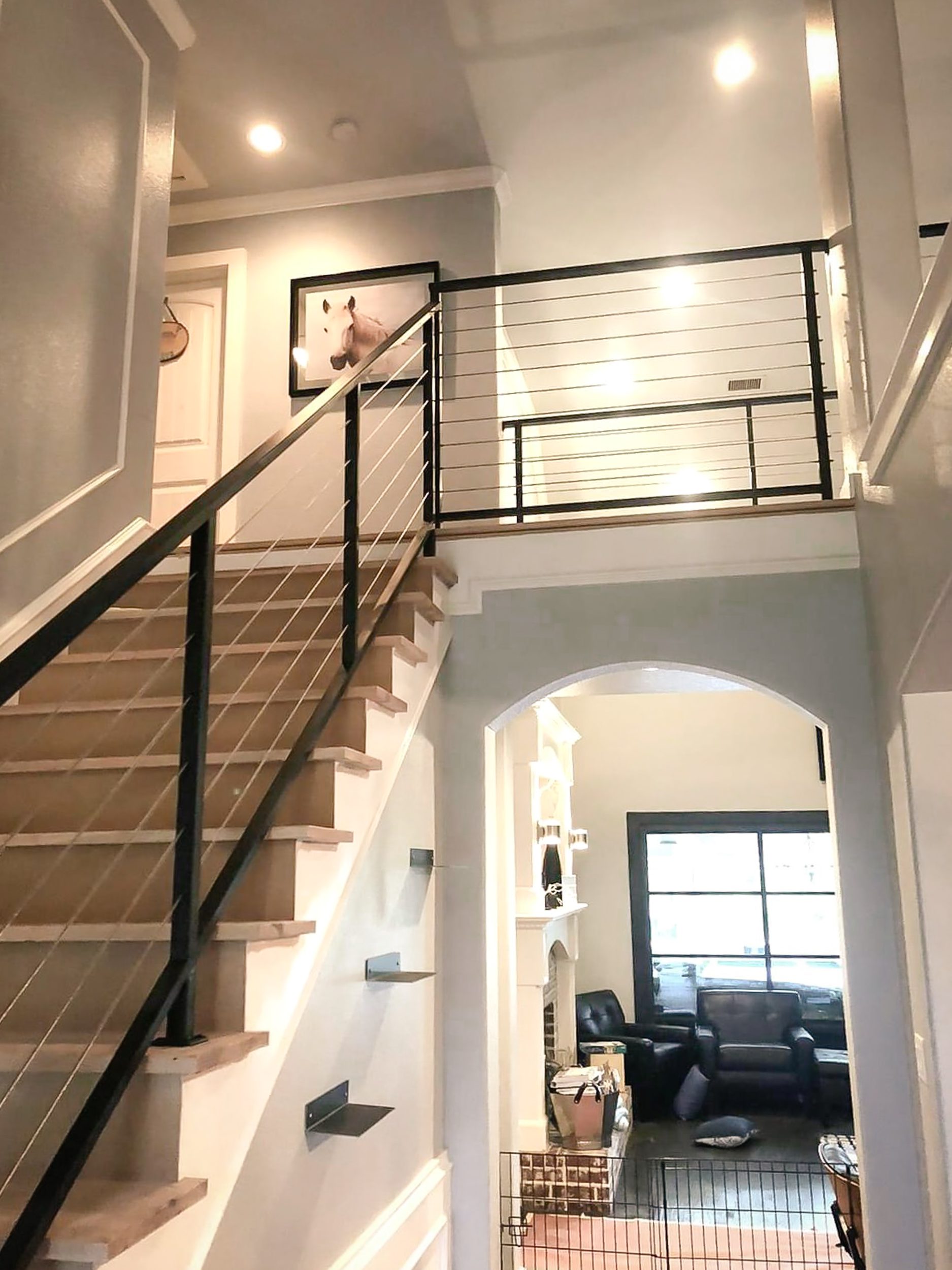This vertically aligned rectangular photograph captures the interior of a house, focusing on a doorway area that leads into various parts of the home. The primary feature on the left side of the image is a staircase with wooden steps and a black metal handrail. The stairs ascend to an upper level illuminated by several lights. On this upper level, a framed picture of a horse adorns the white walls. 

In the foreground, towards the bottom right corner, there's an archway leading into a living room, partially sectioned off by a simple black wire gate resembling a crate gate for animals. Peeking through the gate, the living room reveals charcoal-colored stained concrete floors, leather furniture, and a large window with a black border. A side view of a fireplace can be seen to the left of the living room setup. The consistent color scheme and details, such as the matching black railing and the prominent horse picture, provide coherence to the home's interior design.